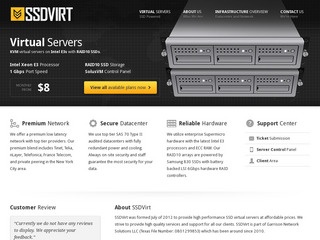A screenshot of a website dedicated to selling virtual servers and server space. At the top, there's a logo featuring the text "SSD VIRT" in white, accompanied by a yellow icon of identical height to the letters, placed to the left of the first 'S'. Although the text on the webpage is blurry, certain details are discernible. One of the promoted virtual server plans is priced at $8. There is a button below this offering labeled "View All Available Plans." The plan specifications, though unclear, mention an Intel Xeon processor, a 1 gigabit port speed, and RAID-configured SSDs. The top section featuring the logo and server ad occupies approximately 35% of the screen.

The remaining 65% of the screen highlights various advantages offered by the service, written in text. These include promotion of a premium network, a secure data center, and reliable hardware. Additionally, there are links to the support center and several customer reviews at the bottom of the page.